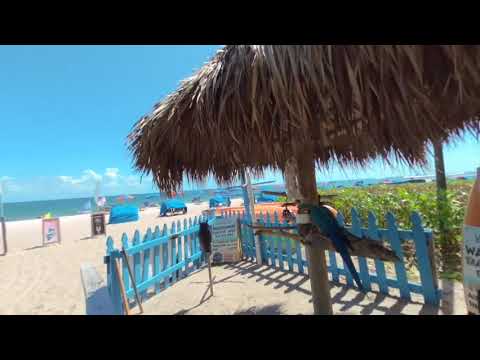This photograph captures a serene beach scene with cream-colored sand extending from the foreground to the horizon. The central focus of the image is a rustic wooden structure resembling an umbrella, made from dried palm fronds and supported by wooden poles. Surrounding this structure is a bright blue picket fence, which includes decorative elements such as oars. Notably, there is a blue parrot perched under the canopy, with a green bird close by, though it appears slightly blurry.

In addition to this focal point, the beach features several bright blue chairs spread out along the sand, contributing to the colorful and inviting atmosphere. Numerous signs are visible across the beach, likely for a nearby restaurant, although their inscriptions are unclear. Beyond the sandy expanse, the crystal-clear, teal-colored ocean water meets a vibrant blue sky adorned with a few low-hanging white clouds on the horizon. The photograph is framed with two black horizontal strips at the top and bottom, emphasizing its detailed yet tranquil composition. The overall scene suggests a sunny, bright day, with sunlight illuminating the sand and casting a warm, inviting glow across the entire beach.